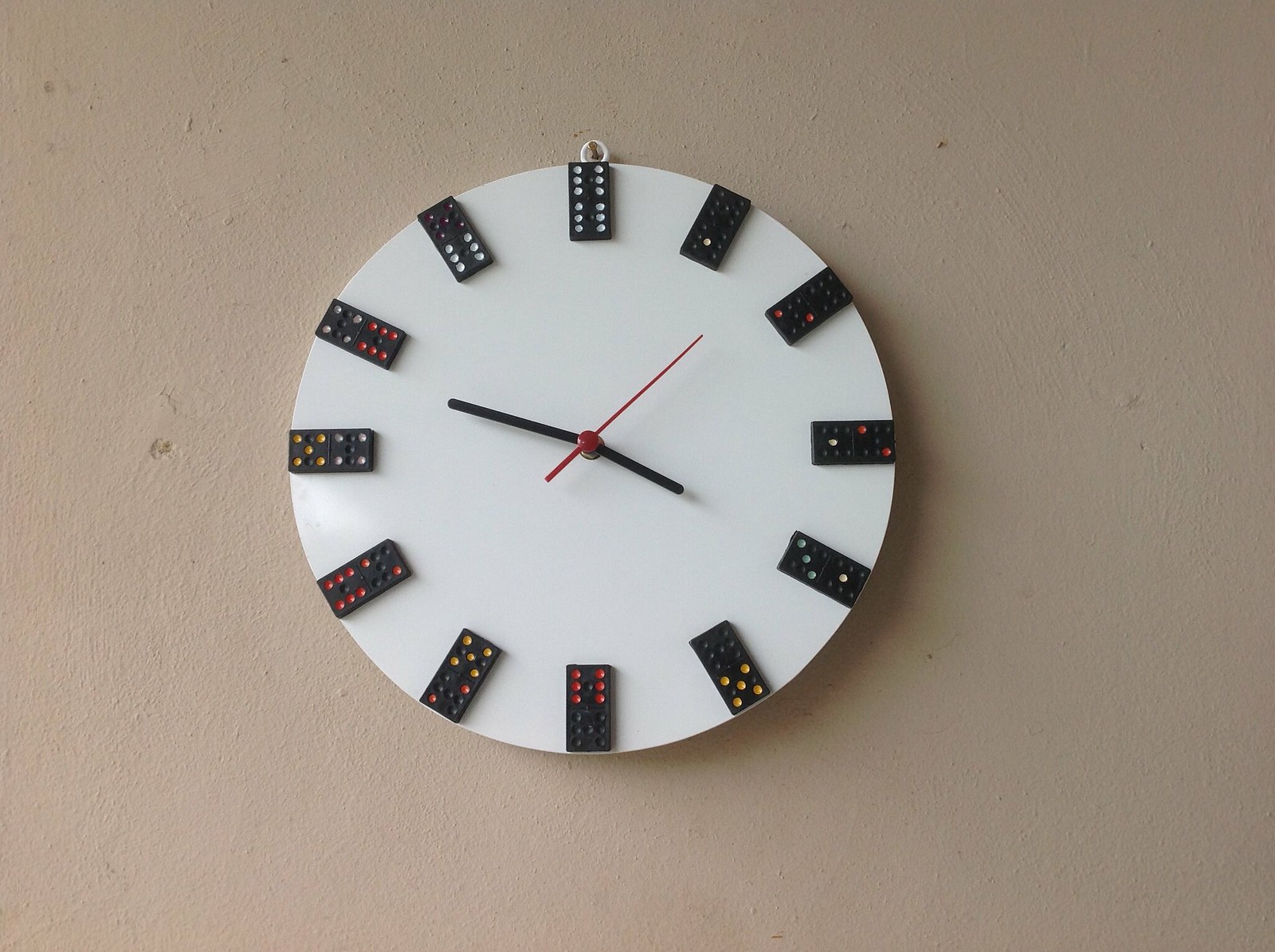This photograph features a distinctive and creative clock mounted on a light beige stucco wall, which shows slight signs of wear and small areas of damage. The clock is quite unique, with a white base and an assemblage of dominoes used in place of traditional numbers. These black dominoes, adorned with red, yellow, and white dots, evoke a vintage feel reminiscent of the 1960s or possibly earlier.

Each domino represents an hour on the clock, starting from the top with the domino for 12 o'clock, which features 12 white dots. Moving clockwise:
- The 1 o'clock position shows a domino with one white dot.
- The 2 o'clock position has a domino with two red dots.
- The 3 o'clock position also has a domino with two red dots and one white dot.
- The 4 o'clock position is indicated by a domino with four white dots.
- The 5 o'clock position displays five yellow dots.
- The 6 o'clock position is marked by a domino containing six red dots.
- The 7 o'clock position features a combination of five yellow dots and two red dots.
- The 8 o'clock position has a domino with eight red dots.
- The 9 o'clock position shows a domino with five yellow and four white dots.
- The 10 o'clock position features a domino with six red and four white dots.
- The 11 o'clock position displays a domino with six white dots, though some dots that should complete the total of 11 are faded or missing.

Completing the clock's design, it has black hour and minute hands, and a red second hand, contributing to its overall vintage yet quirky aesthetic.